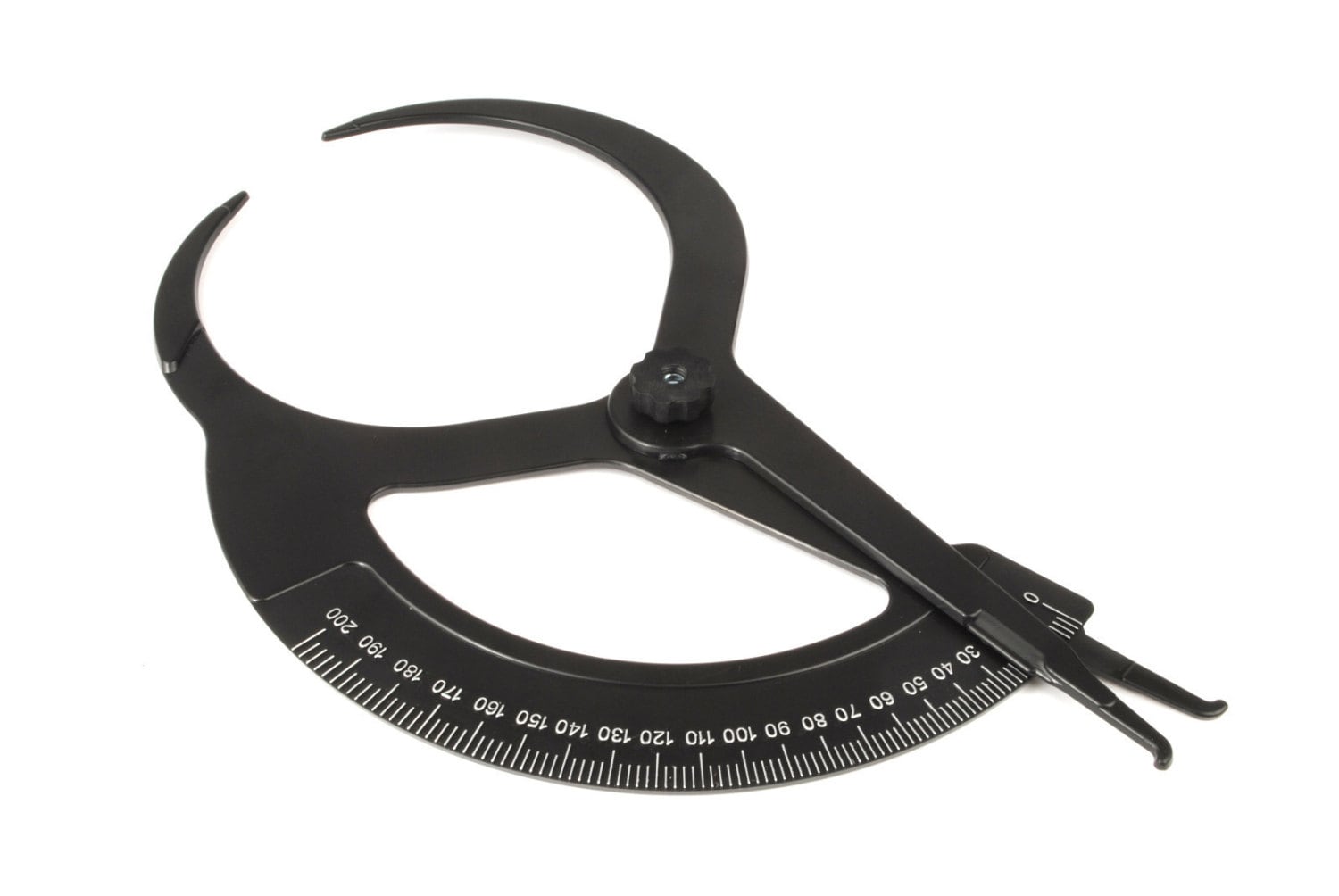The image showcases a black metal measuring tool, likely calipers, designed to measure thickness by opening and closing two metal pieces bolted together. This tool, featuring a sleek black color with white numerical markers ranging from 0 to 200, is set against a solid white background. The clarity of the image is exceptional, aided by natural light that brightens the entire scene. The calipers have curved features toward the upper left, forming an arc, with the numbers starting at the bottom right and curving up to the left. In the center of the tool, a visible screw holds the instrument together, ensuring its functionality. The overall image is free of additional objects, words, or people, focusing solely on the detailed design of the calipers.